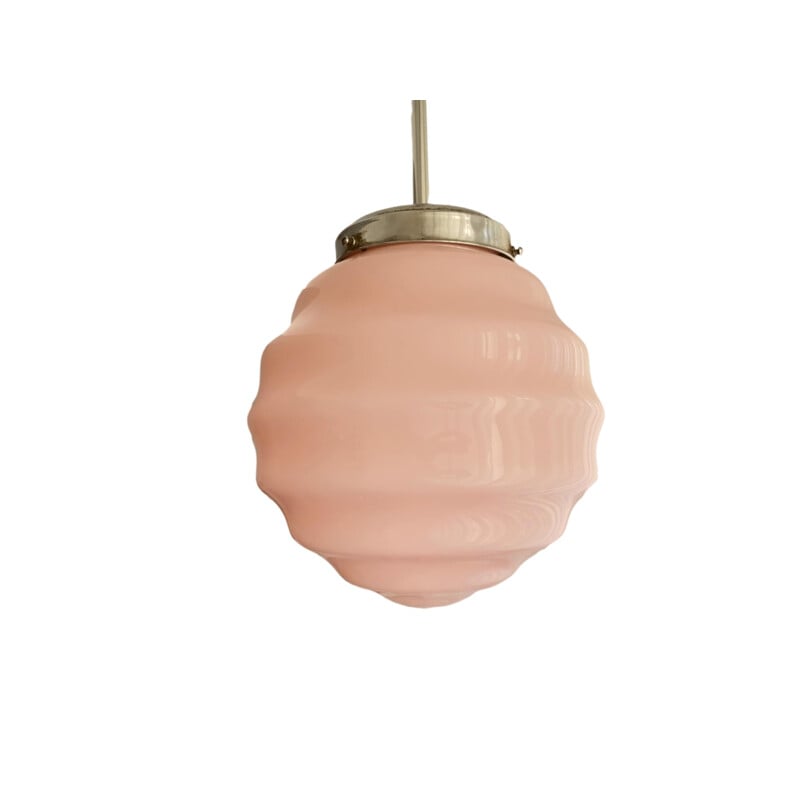This close-up photograph captures an antique hanging light fixture set against an entirely white background. At the top, a silver bar descends to a goldish metal component joined by gray screws in two places. This portion seamlessly connects to a wider section, anchoring a unique, asymmetrical glass bulb that exudes a vintage charm reminiscent of the 1950s. The glass bulb, shiny with a pronounced squiggly and uneven texture, takes on a spherical bowl shape and displays a delicate pinkish salmon hue accentuated with decorative ridges, adding to the fixture's distinct, antiquated elegance.